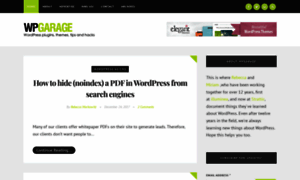The image appears to be a low-resolution, blurry screenshot of a website. The layout includes a prominent black top bar with design elements in lime green. On the left side of this top bar, there is a small lime green square, while the far right features four lime green dots arranged horizontally. Beneath this top bar, set against a predominantly white or gray background with scattered black boxes, is the website's logo in the left-hand corner. The logo reads "WP Garage," with "WP" rendered in black and "Garage" in lime green. In the central part of the image, there is a block of black text that is difficult to read due to the blurriness, but it seems to address a tutorial topic. The decipherable portion of the text indicates that the website provides instructions on "how to hide a PDF in WordPress from search engines."